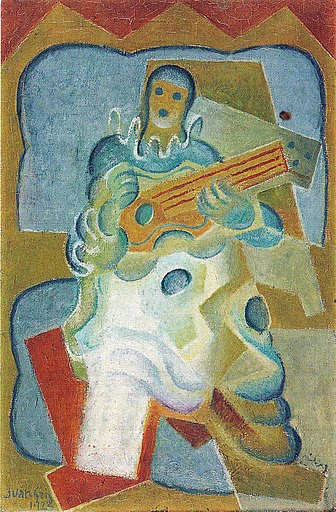The image is an abstract painting featuring a figure that resembles a clown due to its geometric and surreal portrayal. The figure in the center is adorned in a long, fluffy, blue multi-shaped garment with a tall, frilled white collar around the neck. The face is simplified to three blue dots: two representing eyes and one as a mouth, with no discernible nose. The figure's hands and legs are painted in a cool blue, with the legs appearing almost melting, reminiscent of Salvador Dalí's style. 

In one hand, the figure holds a rectangular object adorned with a circle on one side and three red lines on the other, suggesting it might be a guitar. The background is a vibrant mix of abstract shapes and colors including rich reds, earth tones, yellows, and blues. Some of these shapes are reminiscent of an elephant but remain indistinct and abstract, contributing to the painting's overall surreal quality. The background and surroundings are composed of both wavy and angular shapes, further enhancing the painting's abstract nature.